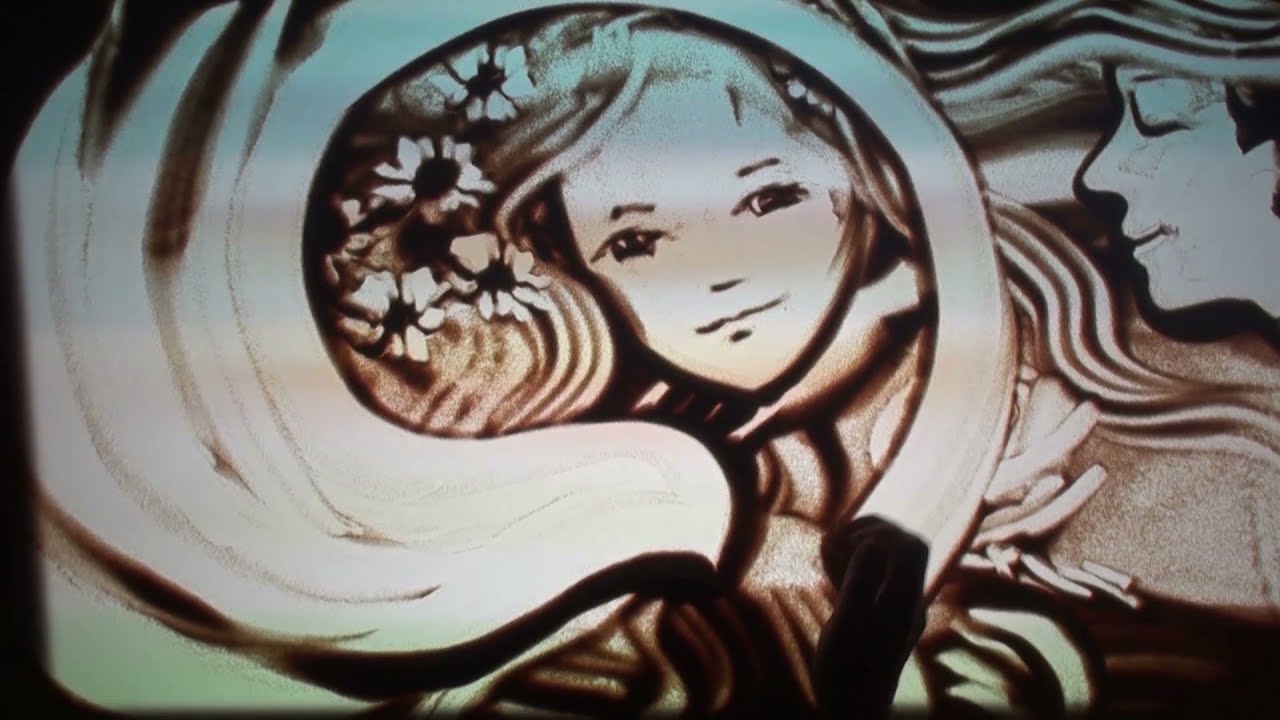This image appears to be a close-up, black-and-white or sepia-toned drawing that features a young girl with long, wavy hair adorned with four flowers. She is smiling warmly and looking directly at the viewer, her face framed by a distinctive swirling pattern that mixes white, black, and faint hints of brown and red. The swirls, which might resemble a swan neck, add an ethereal touch and are lined with 4 to 6 delicate lines. To the right, partially visible, is a man with his eyes closed, smiling softly, as if looking at or leaning towards the girl. The intricate detailing emphasizes the lines in her hair and highlights her sharp chin and small facial features, encapsulating a moment of serene connection between the two figures.